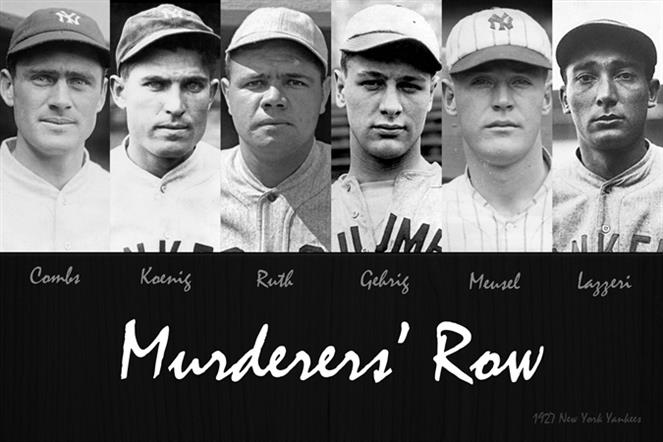The image is a black and white photograph divided into two sections. The top half features six vintage portraits of baseball players from the torso up, all wearing New York Yankees caps and jerseys with varying shades and textures. Each player has a serious to neutral expression. Their names are listed from left to right as Combs, Koenig, Ruth, Gehrig, Meusel, and Lazzeri. Below the portraits, in a cursive white font against a black wood-like background, the text reads "Murderers Row." Positioned in the bottom right corner is the caption "1927 New York Yankees," also in white text.